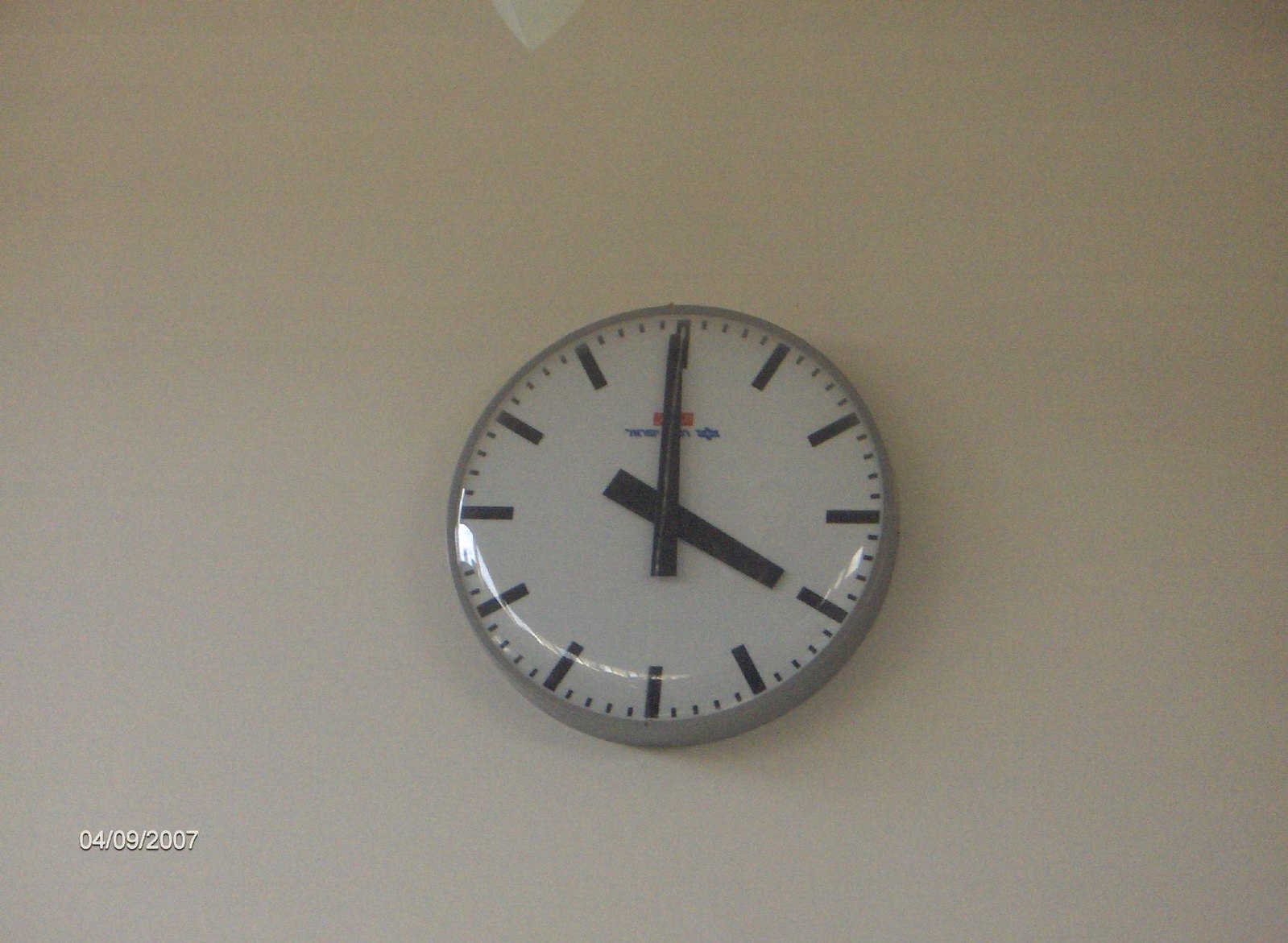A minimalist wall clock is mounted on a plain white wall. The clock face is free of numbers, instead featuring small dashes to denote each hour and larger dashes at the cardinal points of 12, 3, 6, and 9 o'clock. It is currently indicating precisely 4:00, with both the hour and minute hands appearing as thick, rectangular black bars. No second hand is present. The clock has indistinct red and blue lettering on its face, and the date "0409-2007" is printed in small characters on the bottom left, signifying April 9th, 2007.